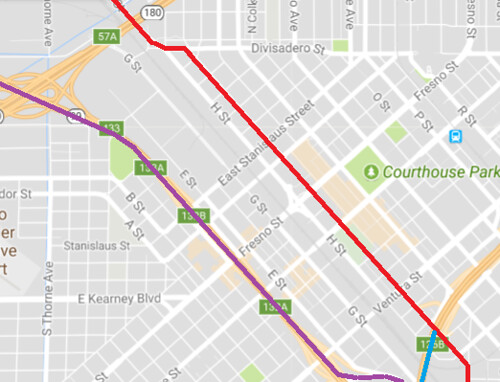A detailed and cleaned-up caption for the described image could be:

"An overhead map vividly depicts the layout of a city, showcasing blocks in gray and roadways highlighted in yellow and white. Two prominent lines, one in purple and another in red, trace a diagonal path from the top left to the bottom right of the map. Various highways, illustrated in yellow, are marked with green rectangular signs featuring their respective numbers. Street names are subtly noted in gray. In the center, Fresno Street traverses horizontally, acting as a notable landmark. A green text indicator, accompanied by a tree icon, marks the location of Courthouse Park. Additionally, a highway number is presented in white text within a black-bordered white oval."